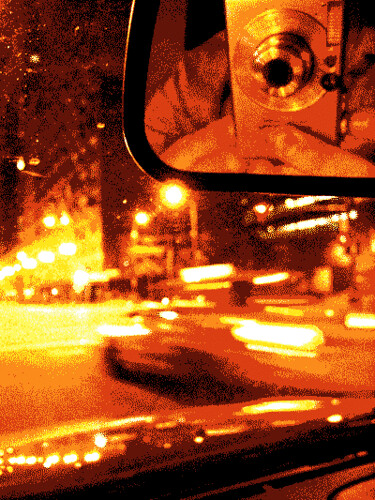In this nighttime photograph, taken from inside a vehicle, we observe the vivid, grainy, and blurry scene through a reddish-brown tint. The main focus is on the reflection in the rearview mirror, where a person is holding a silver camera with an extended lens, capturing the moment. Their fingers grip the bottom of the camera, with their shoulder slightly visible above. The camera, which appears to be more sophisticated than a disposable one, is aimed at the mirror, capturing both the internal and external environment.

Through the windshield, we notice blurred streetlights and the shiny front hood of the car displaying reflections. On the right side of the vehicle, other cars move past, contributing to the blurred effect, implying motion or a slow shutter speed. Further ahead, tall buildings with numerous illuminated windows add a bustling, urban backdrop to the scene. The prominent red and orange hues dominate, reminiscent of fire colors, enhancing the nocturnal and dynamic atmosphere of the photograph.